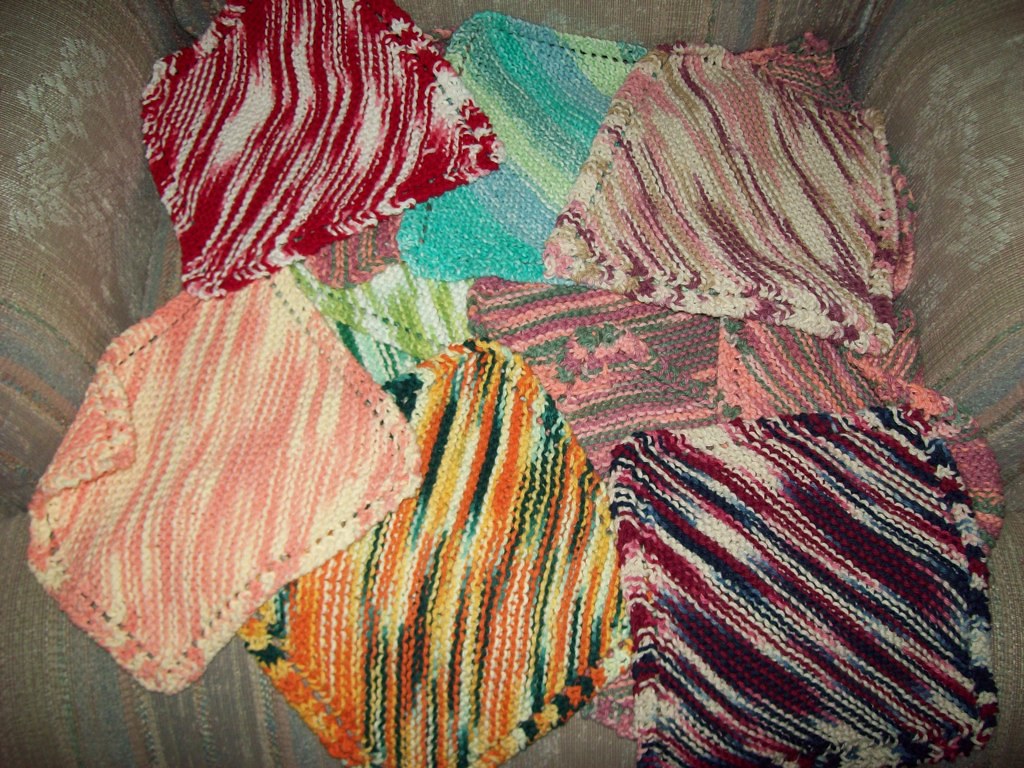The photograph captures a cozy array of a dozen or more knitted dishcloths artfully displayed on an upholstered armchair. The chair is covered in a charming fabric adorned with a floral print and pastel stripes, providing a soft, vintage backdrop to the vibrant knitted pieces. Each dishcloth features a consistent pattern of diagonal stripes, made more dynamic by the use of variegated yarn. They are loosely piled atop one another in the chair, their colors and patterns intertwining in a visually appealing arrangement.

Highlighting the variety, there is a dishcloth that stands out with its vibrant red and white stripes at the top of the pile, slightly off-center. Another dishcloth nearby combines shades of dark green and two tones of orange, creating a striking contrast. A pink and cream cloth adds a softer touch to the mix, while a bold combination of dark red, dark blue, and white invokes a sense of depth. Two of the dishcloths share a similar palette of pink and green, hinting at a cohesive design choice. Tucked within this assortment are also dishcloths in pink, mauve, tan, and cream, along with a pattern combining blue, green, and gray.

The overall composition of the dishcloths in the armchair evokes a sense of comfort and handmade craftsmanship, with each piece contributing to a rich tapestry of color and pattern.